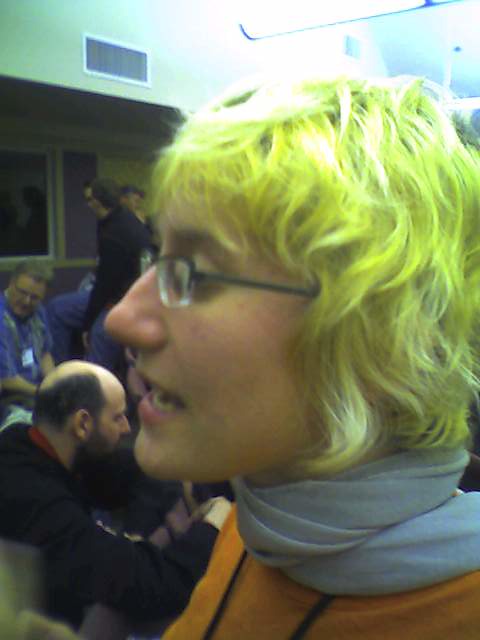This detailed photograph captures a close-up side profile of a young person with medium-length, neon yellow hair styled with sloppy bangs that reach the nape of their neck, evoking a 1960's aesthetic. Their gender is ambiguous, possibly female, as they sport a gray scarf tied in a feminine manner around their neck. They are wearing dark gray, wireframe glasses and an orange shirt adorned with two black strings. This individual also has a lanyard around their neck. The setting appears to be an indoor group gathering, possibly in a meeting venue or a workplace, potentially of a medical nature, as suggested by the presence of individuals in blue scrubs and lanyards in the background.

Behind this person, the room is filled with several people, some seated and others standing. Notable details include a bald man with hair on the back of his head, wearing a black top and sporting a beard and mustache. Nearby, there is another man with sandy hair, glasses, a blue shirt, and an unreadable badge. Additionally, a man in a black shirt and blue jeans stands near the main subject's nose, facing towards the camera. The background features a white ceiling, a purple wall, and a window, adding to the indoor meeting atmosphere. The main subject appears to be speaking to someone, captured mid-sentence with their mouth open.